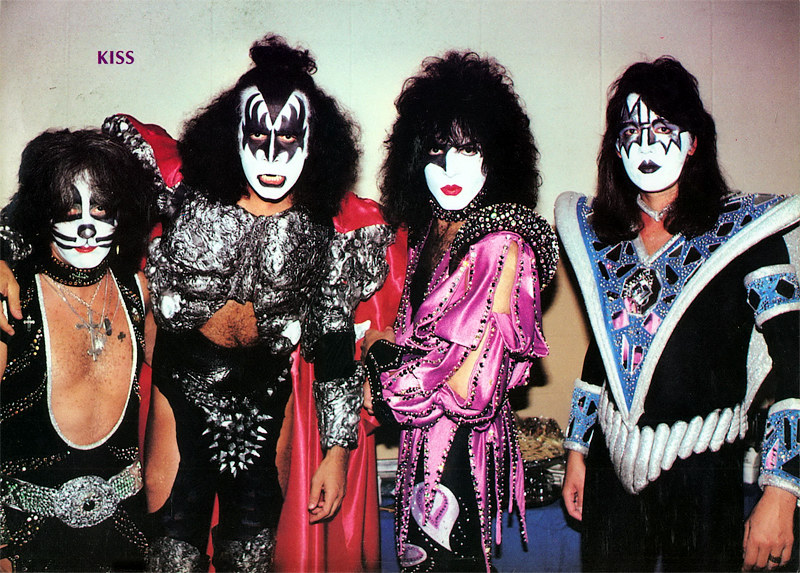In this image, we have the iconic rock band KISS. The band, known for their flamboyant stage personas and elaborate makeup, is set against a white wall with the word "KISS" written in purple in the upper left corner. The four band members, Gene Simmons, Ace Frehley, Peter Criss, and one unidentified member, each sport wild, black, poofy hair and notable face paint designs – including a cat and a star pattern. Their faces are painted white with striking black details and bold lipstick, some in black and some in red. They're dressed in their traditional and extravagant rock-and-roll outfits featuring a lot of black and diamond-studded accessories. One band member is seen with a red cape, another in a purple shirt, and another has a blue piece resembling something an action figure would wear, edged with white borders. This image likely captures the band during their younger years, showcasing their signature look that contributed to their fame.